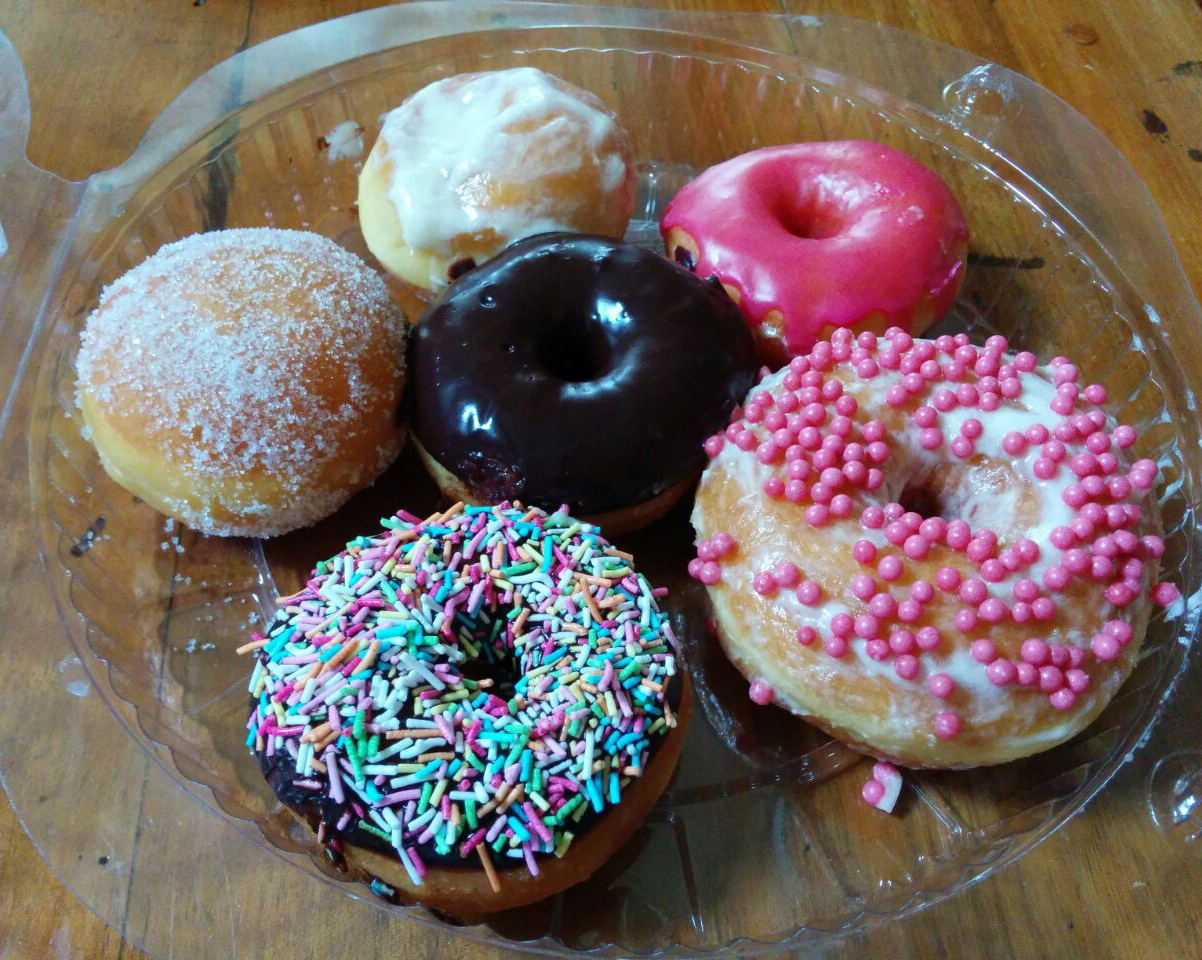In the photograph, a clear circular plastic container with a hinged lid, which is now open, displays six donuts arranged in a pentagon around a central donut. The scene is set on an old, medium-toned wooden table, its rustic surface featuring distinct dark notches and a noticeable stain.

Starting with the central donut, it is a classic ring shape generously coated with smooth dark chocolate frosting. Moving clockwise from the top, the first is a jelly-filled donut covered with a layer of powdered sugar. Adjacent to it is a vibrant hot pink glazed ring donut. Next, descending in the clockwise direction, is a ring donut with a white glaze adorned with light pink bead-like sprinkles, some of which have scattered inside the container. Following this is a chocolate-frosted ring donut decorated with colorful pastel sprinkles in shades of green, white, pink, yellow, blue, and orange. Continuing, there is another jelly-filled donut, simply dusted with granulated sugar. Lastly, positioned between the bottom two but clearly visible in the layout, is a vanilla-glazed donut with a smooth white surface.

The donuts each exhibit a distinct texture and topping, enhancing the visual appeal and making them look fresh and appetizing against the backdrop of the rustic wooden table.